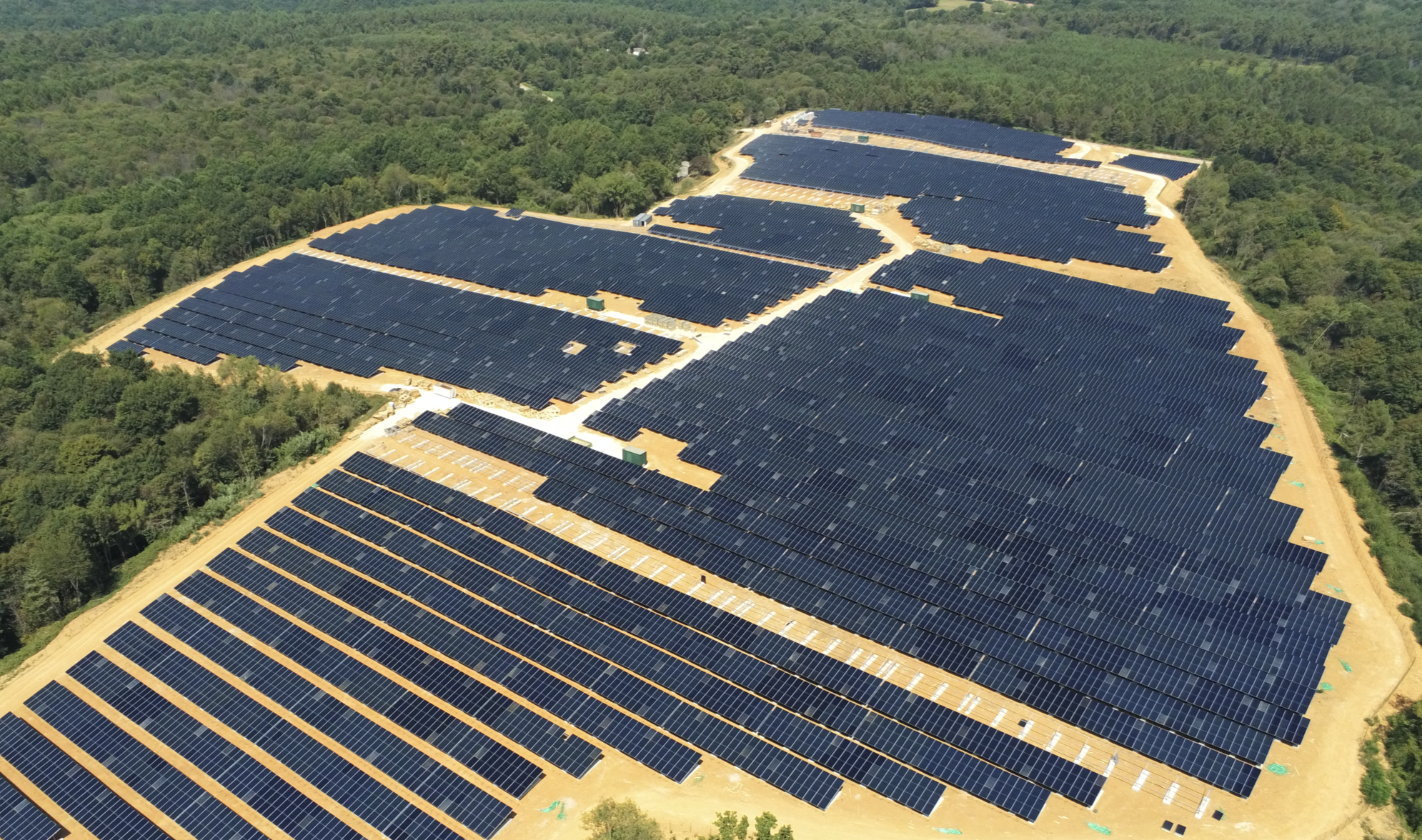An aerial photograph captures a vast solar panel installation set within a thick, lush forest. The field, cleared of trees and greenery, has a yellow, sand-like ground and is triangular in shape, with sections extending into the surrounding dense forest. The solar panels, blue or black, are meticulously arranged in hundreds of rows across the expanse, possibly more than a hundred rows in total. A white path bisects the rows of uncountable panels, providing a stark contrast to the dark, shimmering surfaces. The lush greenery of the forest, brimming with full, verdant trees, envelops the solar panel field on the left, upper, and right edges, emphasizing the harmonious juxtaposition of advanced technology and natural wilderness.